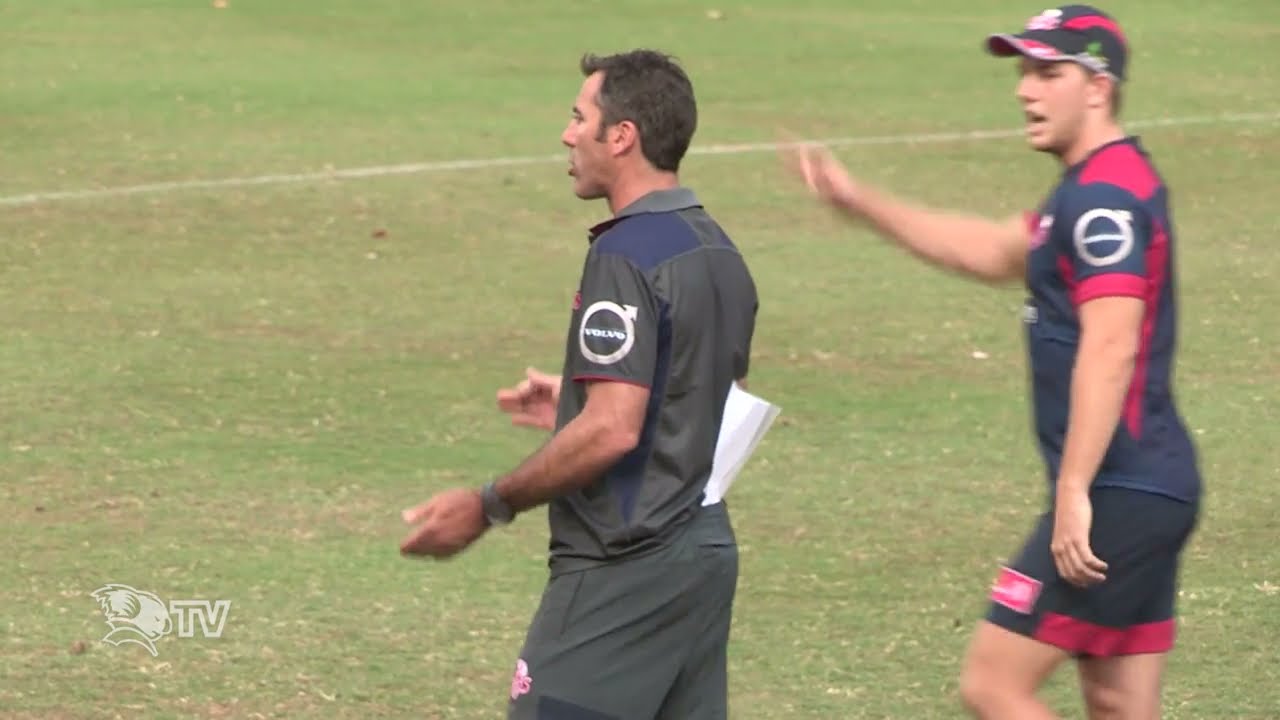This image captures a scene from a training session on a well-manicured soccer field. In the foreground stands a dark-skinned man, possibly a coach or player, poised as if ready to make an athletic move. He wears a navy blue short-sleeve jersey accented with red on the shoulders and sides, adorned with business logos. A red visor rests on his head. Behind him, another man, likely another coach based on his stance and attire, points assertively towards something off-camera. He is a white man with short brown hair, dressed in a collared gray polo shirt and black shorts, also displaying team logos. The setting is an empty soccer stadium with small advertising banners along the walls, including "Brisbane" and "Volvo." The scene is framed by empty rows of pink or red seats rising in the background. A corner watermark with a koala bear logo and the words "Koala TV" is visible in the lower left-hand corner, while the shoulder of another player appears in the lower right-hand corner.